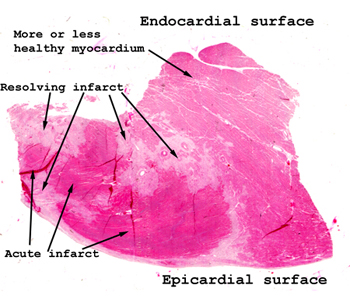The image shows a labeled microscope view of a cross-section of the heart tissue with a pure white background. Central to the image is a pink, rectangular-shaped area with a lobe sticking out the top right. The section displays varying shades of pink and white streaks, resembling the marbling of a steak. The darker pink regions located at the bottom left, bottom right, and the top are annotated with several black arrows and text. The top is labeled "endocardial surface," while the bottom is labeled "epicardial surface." There are arrows pointing to the top right lobe marked "more or less healthy myocardium." Additionally, light pink areas with white holes are marked "infarct," pale pink areas are marked "resolving infarct," and the darker pink section at the bottom left is indicated as "acute infarct." The detailed annotations and various arrows provide specific information about the heart tissue's health and condition.